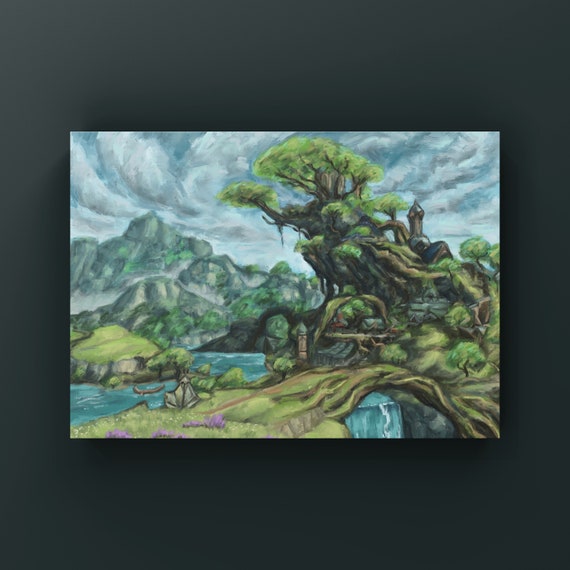This is a photograph of a vibrant watercolor painting, highlighted by a thick black border. The painting portrays a fantastical city, set amidst a lush, forested landscape with whimsical elements. Prominently, a grand old-growth tree with a striking appearance dominates the right side, growing from a cliff overhang and housing a quaint dwelling with a peaked blue roof. Below, a waterfall cascades beautifully, with a bridge crossing over it, leading to a serene lake on the left. The forested hills and mountains in the background add depth and texture to the scene. Towards the bottom left, a small brown canoe rests in the water, near what appears to be a statue of a figure in a lotus position, adding to the painting's mysterious ambiance. The sky above is filled with swirling white and light gray clouds, enhancing the mystical and serene atmosphere of this enchanting landscape.